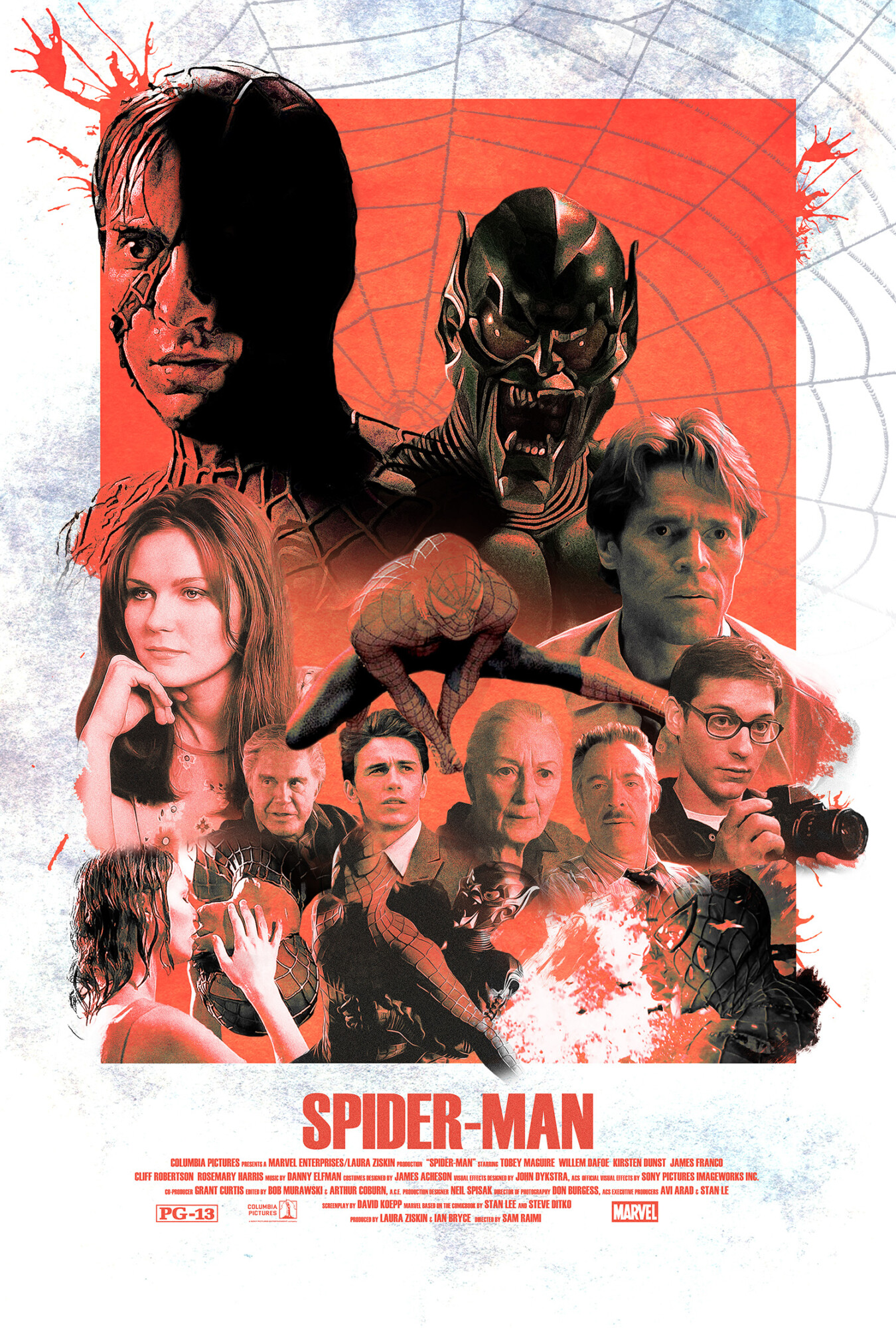This is a detailed movie poster for the film Spider-Man. The poster, predominantly red, displays a striking spider web pattern as the background. At the top left, a partially unmasked Spider-Man, portrayed by Tobey Maguire, reveals part of his face, while prominently featured in the center is the Green Goblin, a menacing figure with pointy ears and golden eyes. The entire image is a montage of characters from the movie, superimposed over a large red rectangle. Along the bottom of the poster, "Spider-Man" is written boldly in red font. Additional details include listings of the main cast: Tobey Maguire, Willem Dafoe, Kirsten Dunst, James Franco, Cliff Robertson, Rosemary Harris, and others. The poster indicates the film is rated PG-13 and is produced by Columbia Pictures in association with Marvel and Sony Pictures.